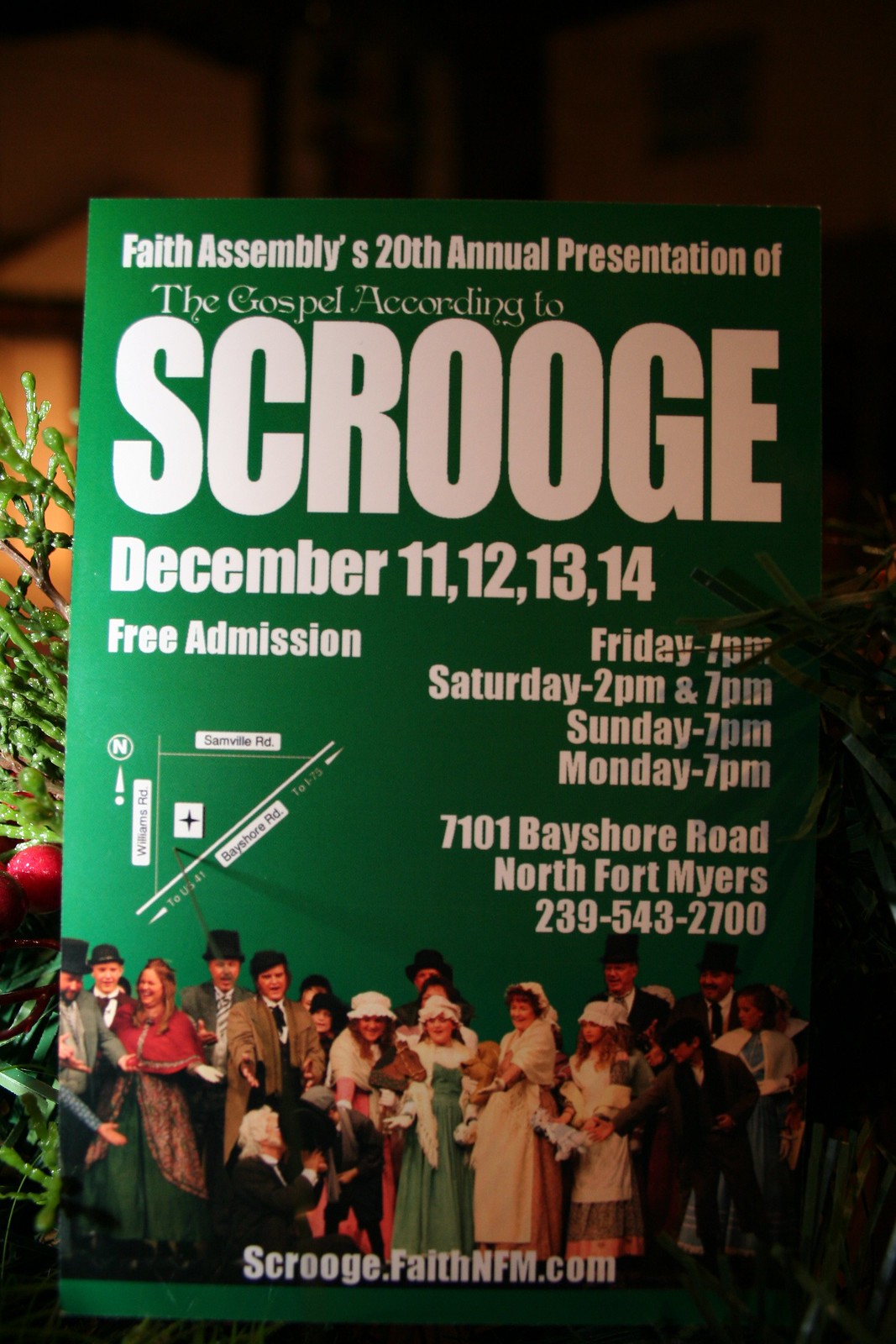The image is a tall rectangular advertisement poster for a theater event, set against a backdrop of green and red Christmas decorations, with a dark upper background. The poster itself has a bright green background with gradient shades, featuring bold white text at the top that reads "Faith Assembly's 20th Annual Presentation of The Gospel According to Scrooge." The poster outlines event details in medium-sized bold text, listing the dates as December 11, 12, 13, and 14, with free admission. Performance times are scheduled for Friday at 7 p.m., Saturday at 2 p.m. and 7 p.m., Sunday at 7 p.m., and Monday at 7 p.m. The location is given as 7101 Bayshore Road, North Fort Myers, with the contact number 239-543-2700. A small map indicating the theater's location is positioned on the middle left. At the bottom of the poster is an image of the cast dressed in period costumes, alongside the website "faithfnfm.com" in white text.